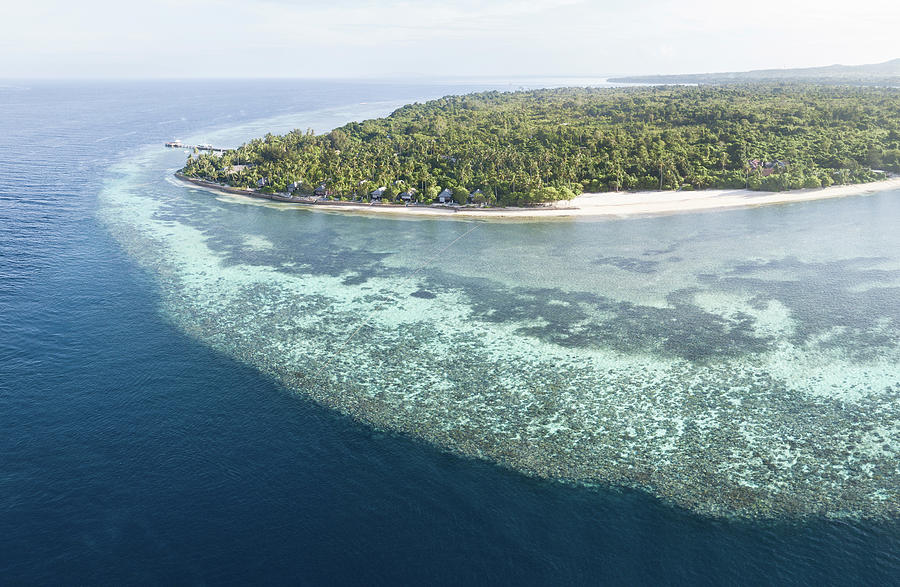This aerial photograph, likely taken by a professional during the daytime using natural light, captures a lush, verdant peninsula extending into clear blue seawater, though it might also be a lake due to its vibrant hue. The coastline of this peninsula is dotted with dense, green trees and flanked by a white sand beach. The clarity of the water reveals a gradual color transition from light blues and greens near the shore, possibly due to the presence of algae or pine pollen, to a deeper blue as it descends. This area showcases underwater features such as coral reefs, sand, and rocks. A small dock is visible, stretching out from the peninsula into the water. The background reveals more landmass under a sky that meets the water in a bright, white horizon, suggesting distant clouds. The island or peninsula appears undeveloped, emphasizing its natural beauty and untouched landscape.